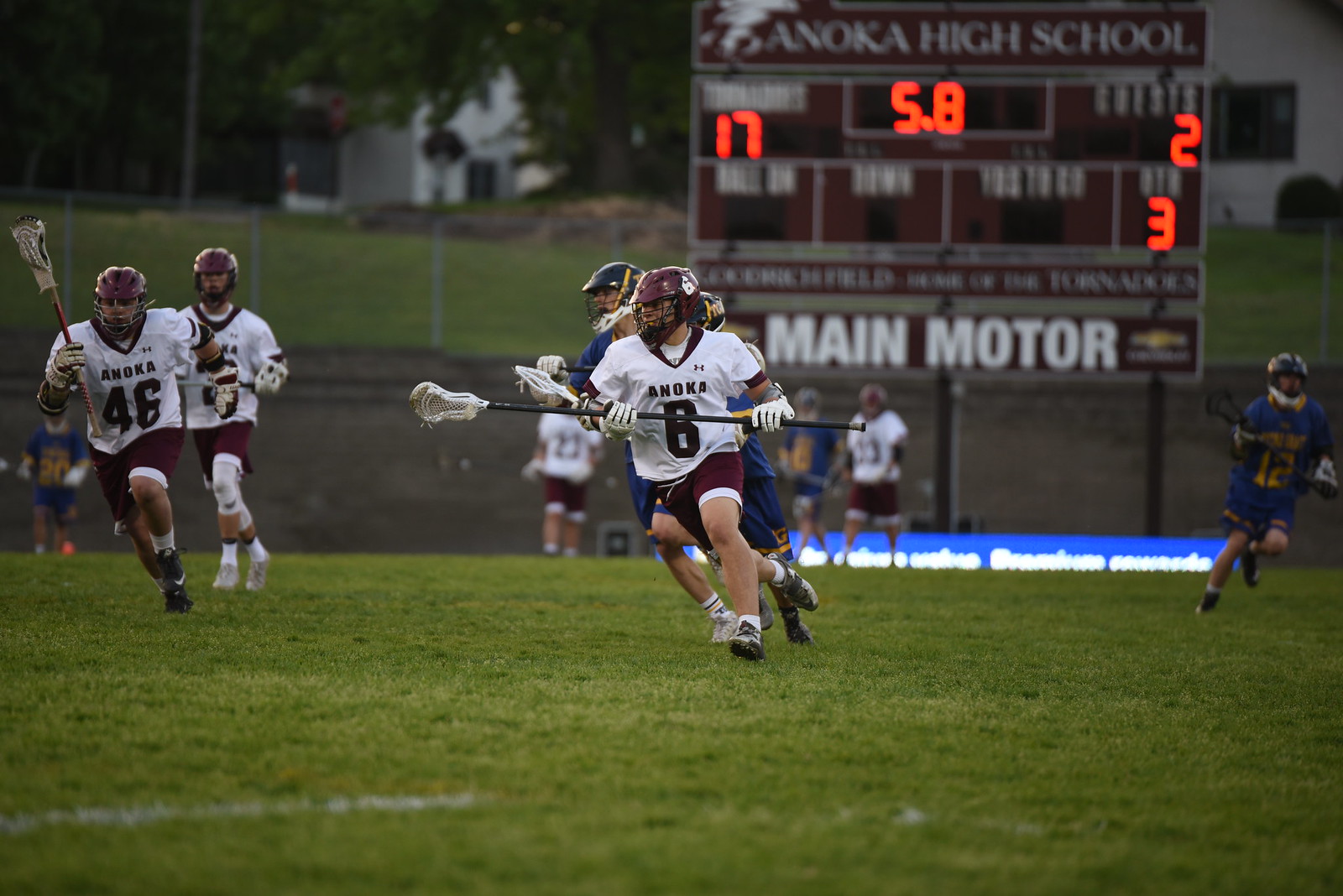In this image, we see an intense high school lacrosse game taking place on a lush green field bordered by a chain-link fence. The scene features 9 players actively engaged, with one team donning white jerseys paired with maroon shorts and helmets, while the opposing team is dressed in blue pants and shorts, accented by blue and yellow helmets and writing. 

Prominently displayed in the background is a large scoreboard labeled "Anoka High School," showing that the home team, Anoka, is leading with 17 points while the guests have 2 points. The scoreboard also indicates there are 5.8 seconds remaining in the third quarter, with "Main Motor" as a notable sponsor featured in large white letters at the bottom. Residential houses and a few scattered trees frame the background, completing the setting of this dynamic high school lacrosse match.